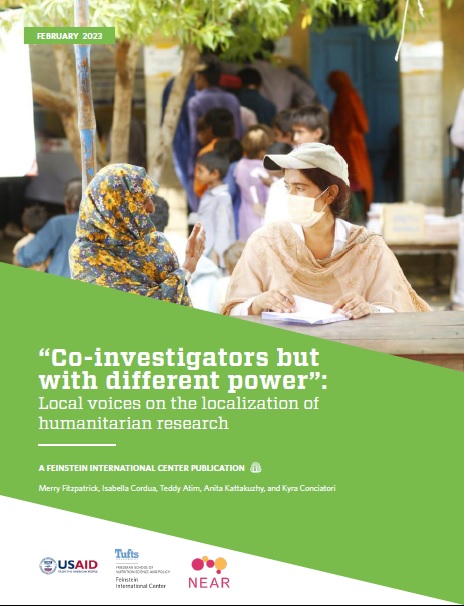This image, dated February 2023, captures a poignant scene featuring two women engaged in conversation. The woman on the right is adorned in a traditional outfit, covering her face with a mask and wearing a baseball cap. Her companion, to the left, is wrapped in a traditional scarf that delicately drapes over her head and body. They are seated at a table, attentively examining some papers.

In the background, a group of children can be seen, along with other women who also have their heads wrapped in scarves, standing under a tree. The setting appears serene yet focused, suggesting a collaborative and communal atmosphere.

Overlaying the image is a lime green section with the text, "Co-Investors, but Different Power." Below it, in white space near the bottom of the image, further details are provided: "Local Voices on the Localization of Humanitarian Research," indicating it is a publication by the Feinstein International Center. The credits list all contributors involved. Additionally, logos for USAID, Tufts University, and NEAR—depicted in pink bubbles with accents of pink and yellow—are prominently displayed.